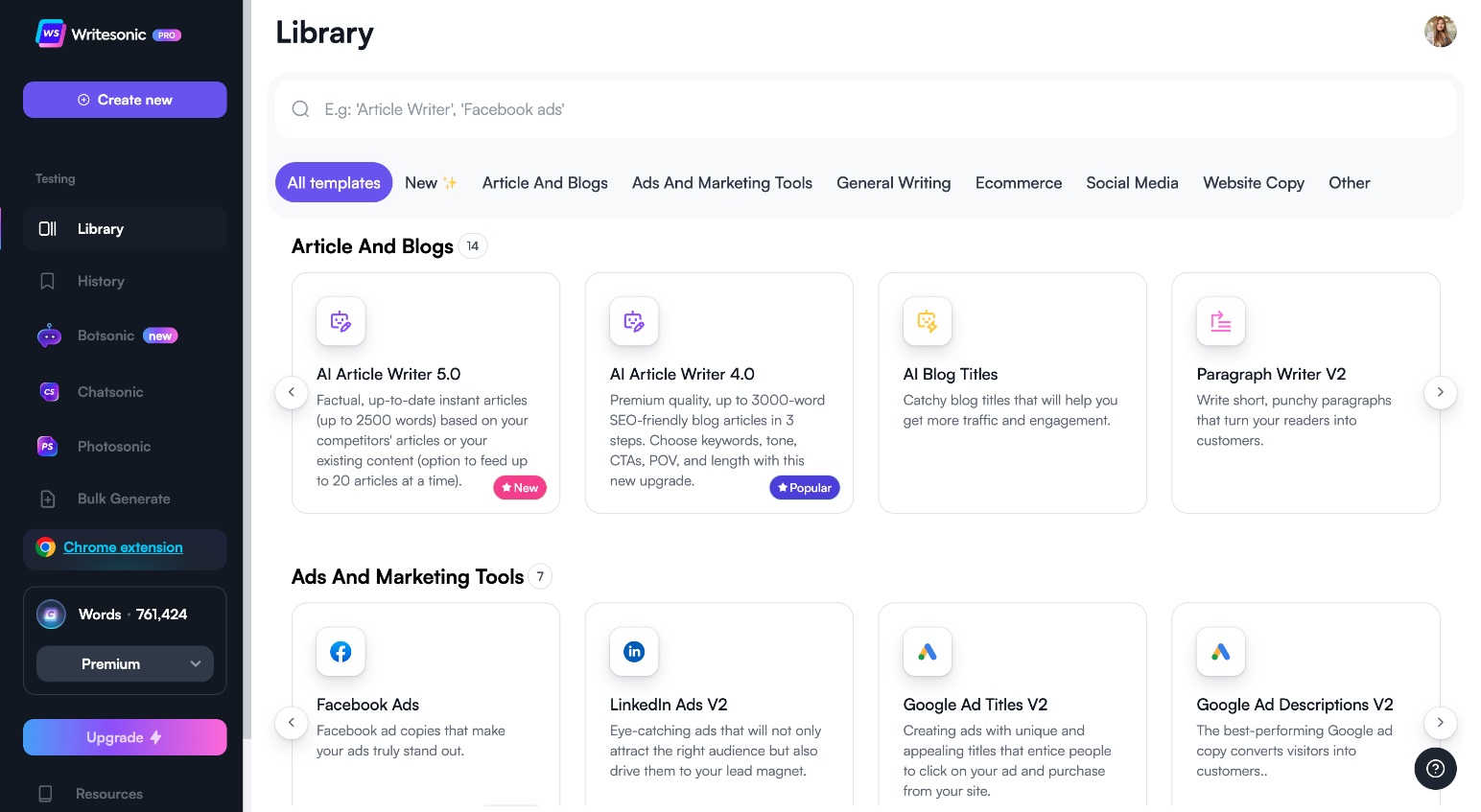The screenshot displays an online-based application interface with a clear division between the left and right sections of the window. The left vertical frame, characterized by a black background adorned with purple and white buttons and icons, serves as the application's navigation panel. This colorful sidebar contrasts sharply with the remainder of the window, which features a white background. 

In the upper left corner of the white section, the word "Library" is prominently written in black. Just below this header, a smaller, dark gray text reads "E.G. Article Writer Facebook Ads." Further down, a purple oval highlights the "All Templates" option, followed by a series of categories labeled "New," "Article and Blogs," "Ads and Marketing Tools," "General Writing," "E-Commerce," "Social Media," "Website Copy," and "Order." Beneath these categories, several articles and blog entries are displayed, although their specific contents are not detailed in the description.

This meticulously organized layout facilitates easy navigation through various templates and writing resources available within the application.